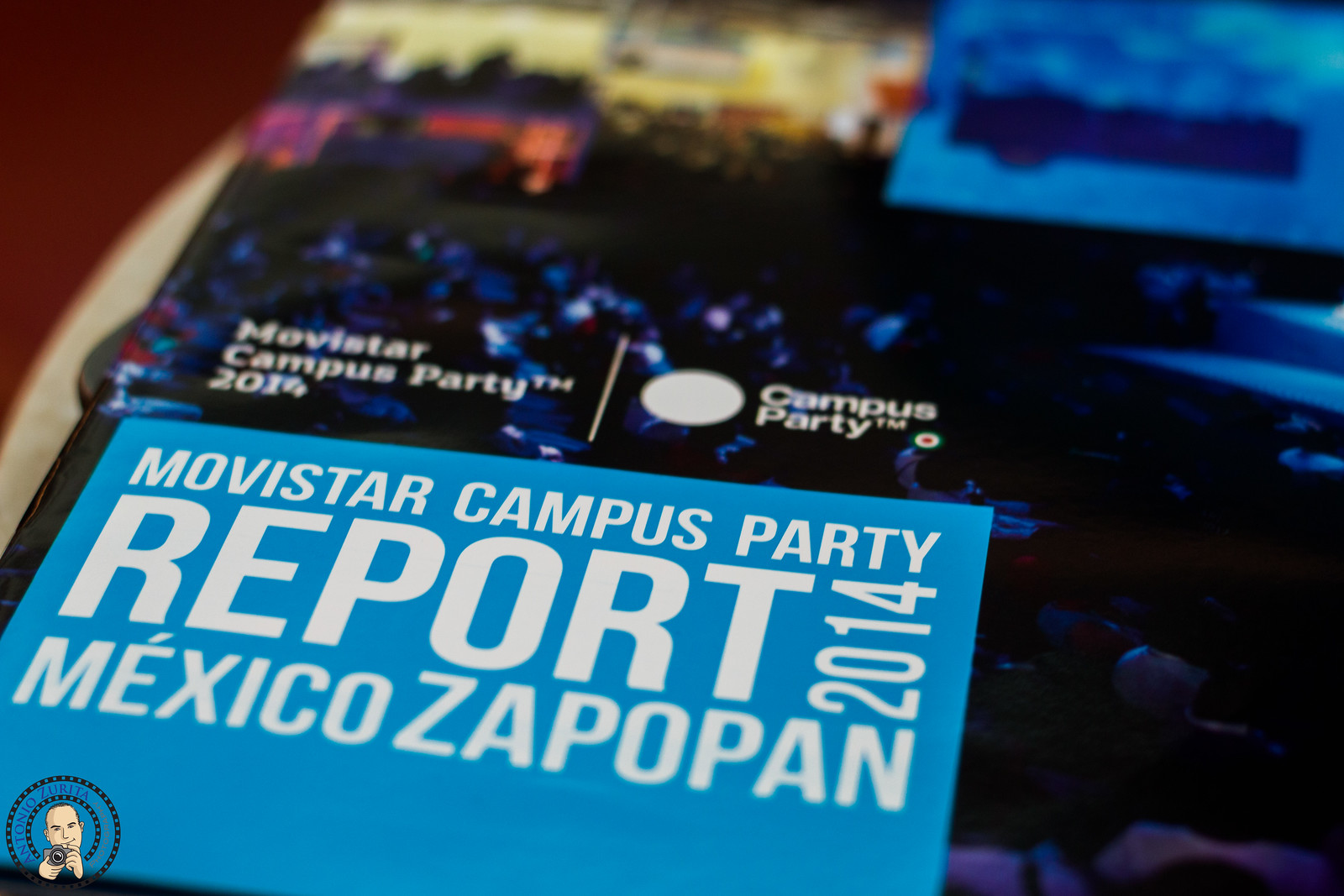The image depicts a vibrant event program or poster, placed on a white table with a glimpse of a red carpet in the background. Dominating the lower half of the image is a striking sky blue rectangular box featuring white text that reads "Movistar Campus Party Report, Mexico, Zapopan, 2014." Above this, smaller white text states "Movistar Campus Party 2014," albeit somewhat harder to discern. To the right, there is a clearer, repeated "Campus Party" text. The background of the poster showcases a blurred audience, likely seated in an auditorium with blue lighting illuminating the space, hinting at a stage or screen ahead. In the lower left corner, an illustration of a man holding a camera is encircled by a black ring, with the text "Antonio Zerita" or "Antonio Zurita Photography" accompanying the logo. The overall image exudes a colorful and energetic vibe with shades of maroon, cream, yellow, red, orange, and multiple hues of blue, suggesting the lively atmosphere of the Campus Party event.